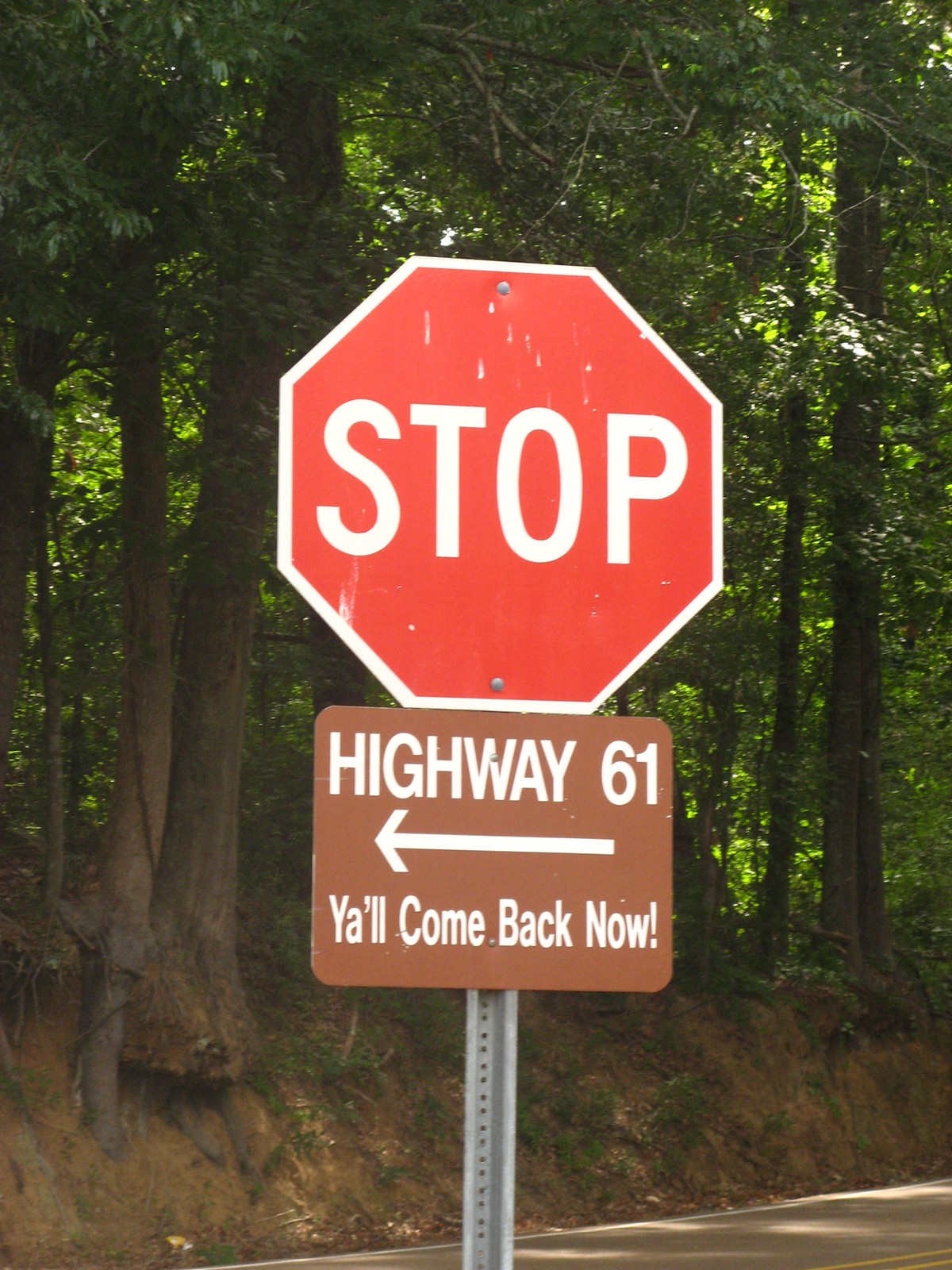In this image, we see a primary focus on a standard red, octagonal stop sign with bold white lettering. Mounted on the same post, just below the stop sign, is a rectangular brown sign bearing the inscription "Highway 61" along with a long arrow pointing to the left. Beneath this designation is a friendly message in white letters: "Y'all come back now." The lower edge of the image captures a glimpse of the road, showcasing a small section of a double yellow line in the bottom right-hand corner. The background reveals a gentle hill leading into a dense forest brimming with greenery, featuring a few tall trees prominently in the foreground while hinting at the lush foliage beyond. The setting suggests a serene, rural environment, possibly within a forested area or a park.